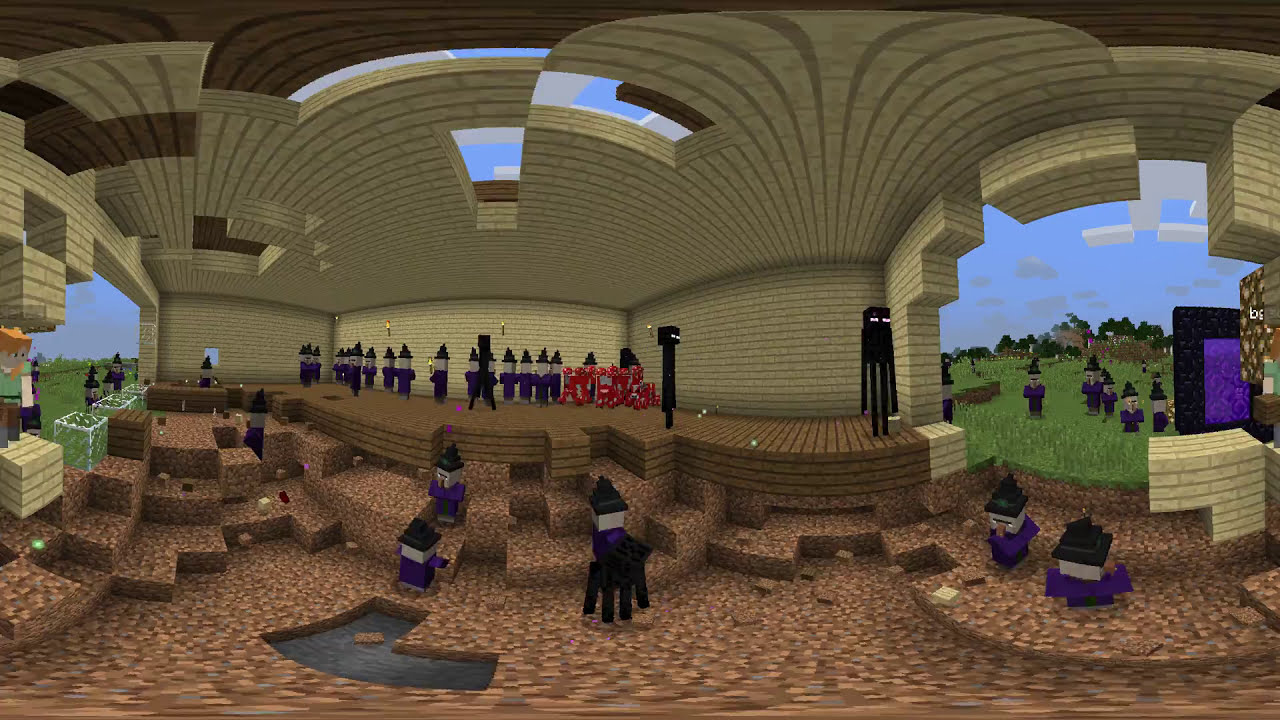The animation depicts a fantastical, open-roof building that lies within a larger structure. The building's notable roof openings reveal a clear blue sky with scattered, block-like clouds. This environment creatively mimics a video game aesthetic with Lego-like features. At its center is a stage, accessible by uniquely cut, cobblestone-like steps. The stage is populated by humanoid figures resembling boxy, Lego creatures—some standing, some seemingly marching in blue uniforms. Moreover, some figures appear to be mounted on animal-like constructs. The subdued, traditional roofing and walls ascend to meet vents that enhance the illusion of an outdoor setting, allowing glimpses of the azure sky. The scene is grounded by a brown and white checkerboard floor which extends to grass-covered outdoor areas where more boxy, soldier-like figures are scattered. Together, these elements create an intriguing, whimsical environment that feels part fantasy and part video game.